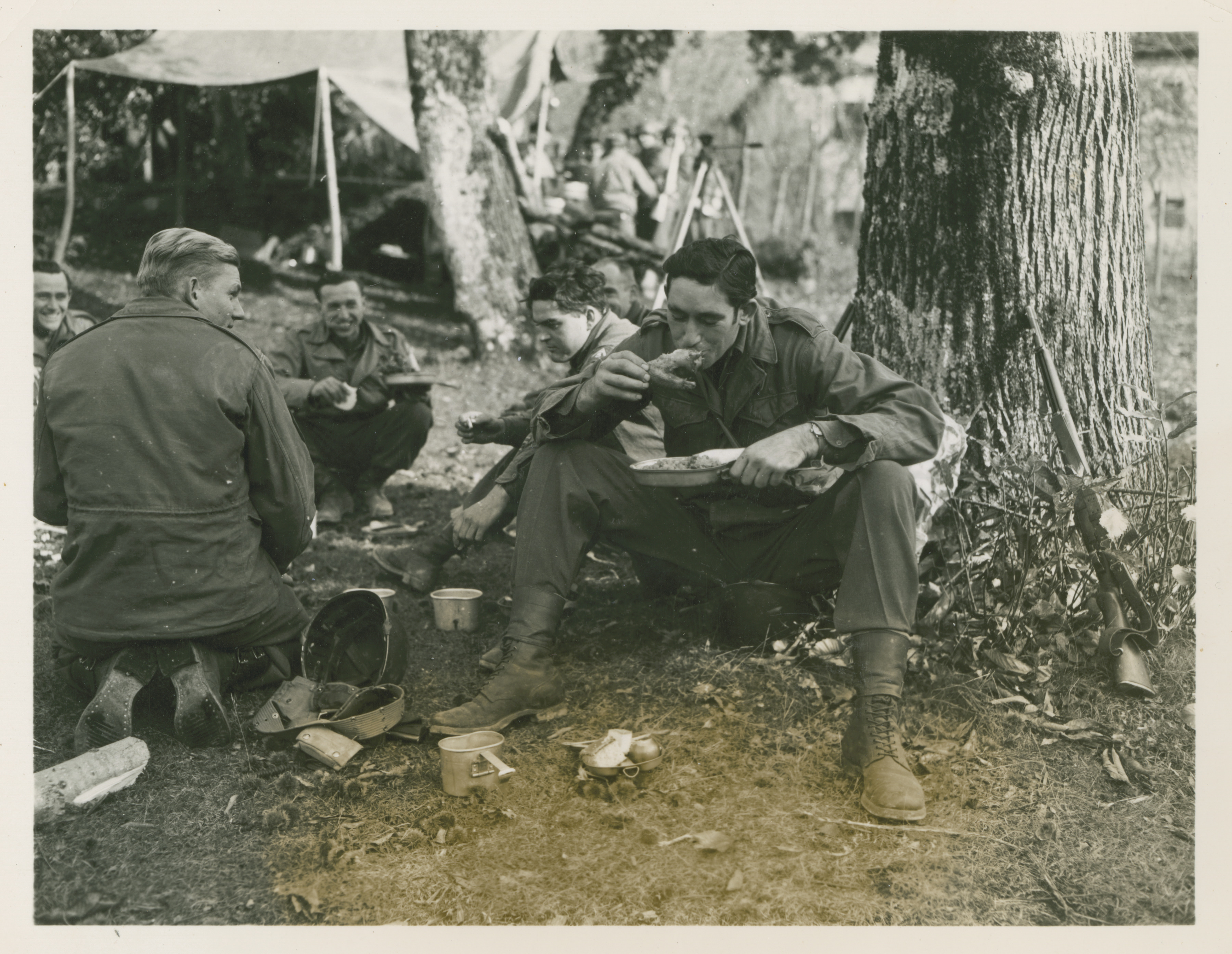In this detailed black and white photograph taken outdoors, three men, likely soldiers, are seen sitting on the ground beneath a large oak tree, engaged in eating a meal. The central figure, a Caucasian man with short brown hair, is leaning against the thick tree trunk. He is dressed in a dark military-style uniform, complete with long sleeves, long pants, black work boots, and a watch on his left wrist. He holds a metal tray or pan in his left hand and appears to be eating with his right hand. Leaned against the tree beside him is a rifle, further suggesting a military setting.

To his right, another man with blondish-brown hair, also dressed in a similar dark uniform, is kneeling and watching the man eating. A third man sits behind them, partially obscured but visible enough to notice that he too is wearing the same style of uniform and boots. He appears to be holding a plate on his lap and laughing, adding a sense of camaraderie to the scene.

In the background, a large tent with poles drapes to the right side of the image, surrounded by other trees whose trunks are also visible. Other figures can be seen walking around the tent, and some men seem to be looking through a telescope, adding to the military atmosphere. The overall scene captures a moment of rest and nourishment for these soldiers amidst their duties.